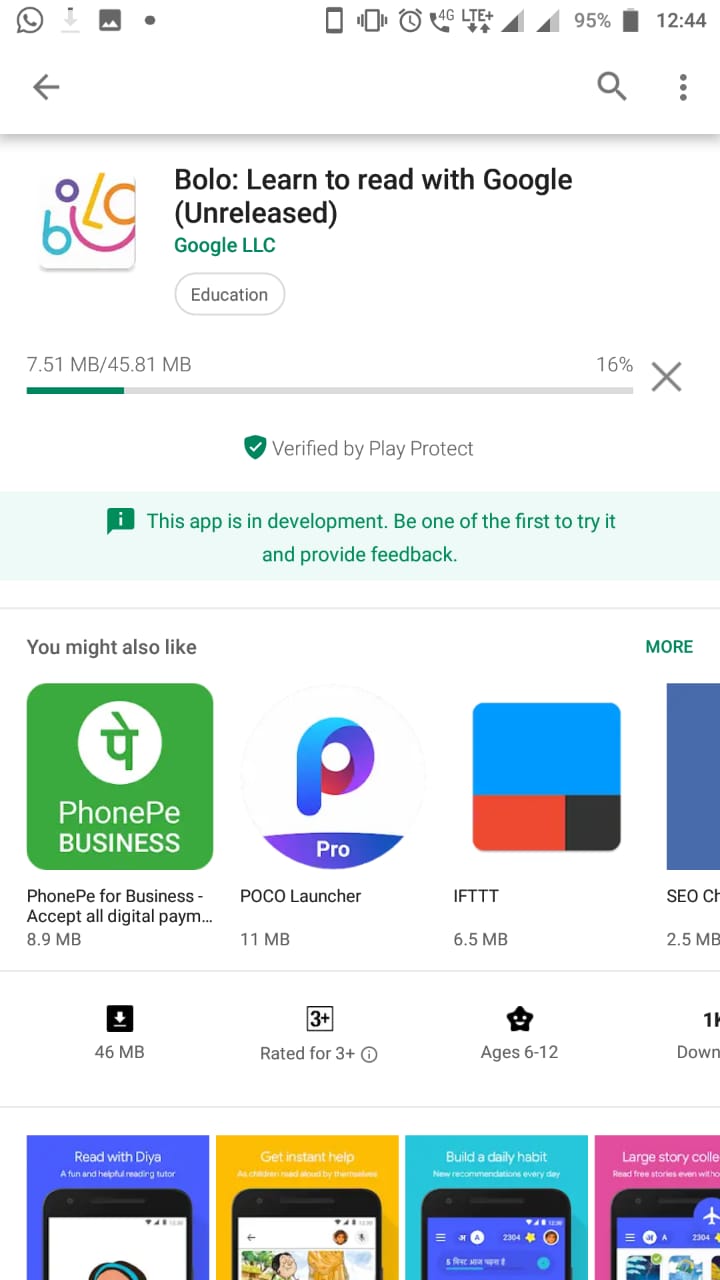The image is a screenshot of a smartphone displaying the Google Play Store page for the app "Bolo: Learn to read with Google," which is currently in the process of being downloaded. At the top of the screen, various status icons are visible, including the signal strength, Wi-Fi, battery at 95%, and the time showing 12:44. Below these icons, there is a search bar and a three-dot menu. The app "Bolo" is categorized under education and developed by Google LLC. The app is labeled "Unreleased," indicating that it is still in development. The download progress is shown as 7.51 MB of 44.81 MB, equating to 15% completion. Below the app description, there are a few suggested apps, including "Phone P Business," "Poco Launcher," and "IFTTT," with one recommendation partially cut off. Due to the small print, the advertisements at the bottom of the screen are not legible.